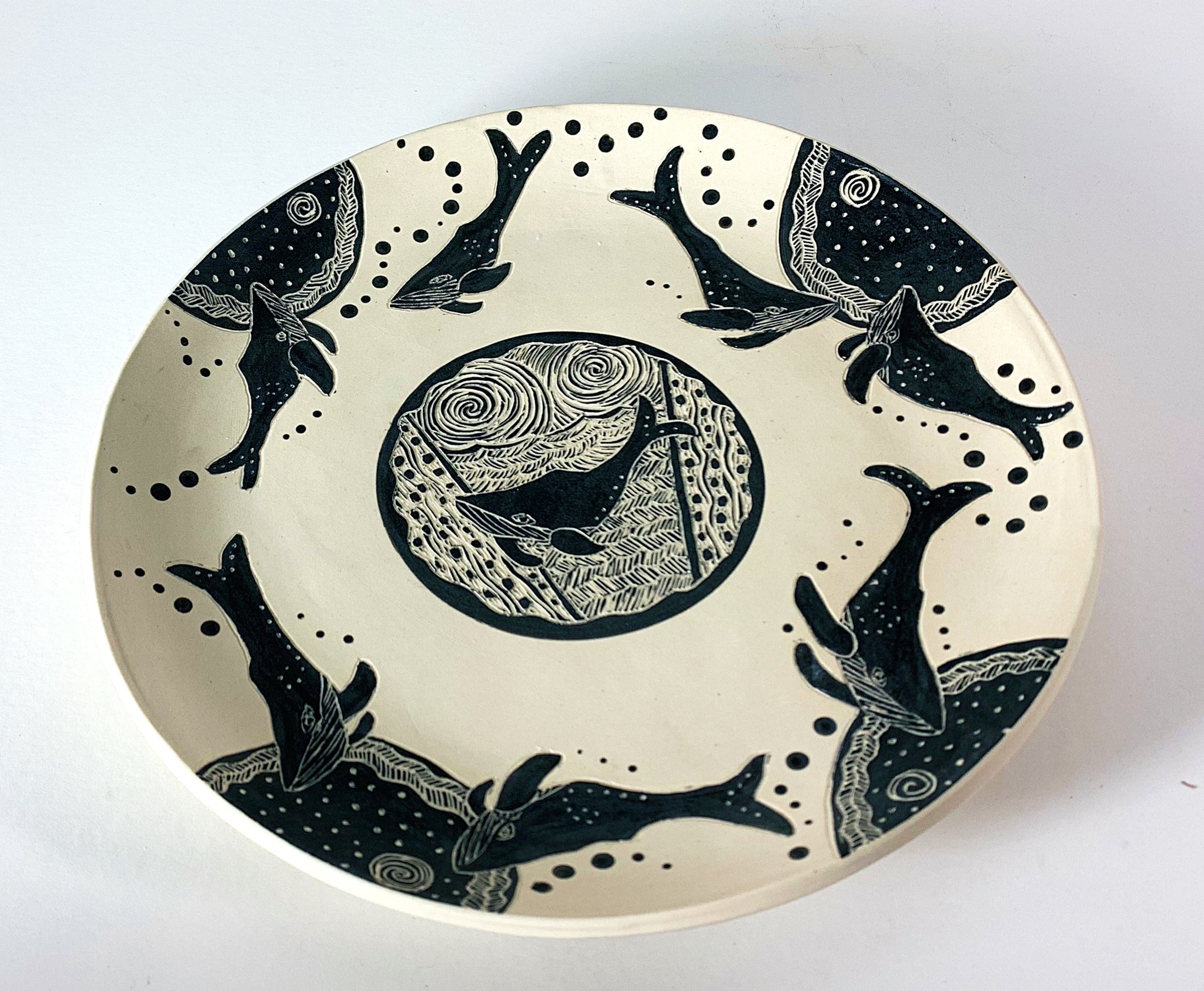The image showcases a circular, handcrafted clay plate set on a white tabletop with lighting casting shadows and highlights across the surface. The plate is an off-white or beige color with intricate black etchings and designs. At the center of the plate is a black circle featuring a detailed depiction of a humpback whale, surrounded by swirly, wavy patterns meant to resemble water. Diagonal lines with black dots create a visually textured backdrop within the circle. Surrounding the central design are repeated smaller etchings of humpback whales along the border, interspersed with black dots resembling bubbles. Additionally, four half-circle designs adorned with white dots and seaweed-like patterns intersect the outer ring of whales, further enhancing the detailed craftsmanship. The gray background of the image, coupled with reflections and glares, suggests a well-lit setting, potentially from the left side, where the light source creates varying shades on the plate and its surroundings.